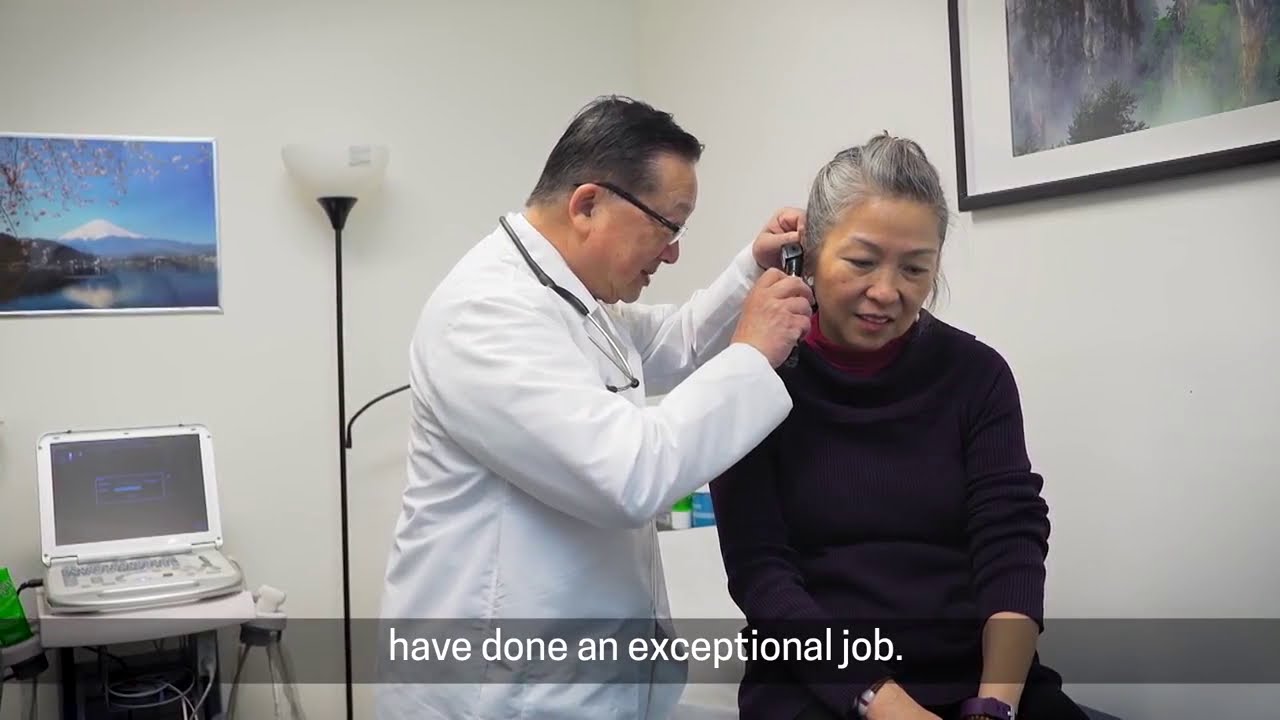The photograph captures a detailed scene in a doctor's office, where an older Asian woman with gray hair, styled in a French braid, is being examined by an Asian doctor. The doctor, who has dark hair with some baldness, is wearing a long white coat and has a stethoscope around his neck. He sports black eyeglasses and is closely inspecting the woman's left ear with a small medical device. The woman, seated on an examination bed, is dressed in a long-sleeve black sweater with the sleeves pulled up to her forearms, revealing that she is possibly wearing a watch. 

To the left of the doctor stands a tall black and white floor lamp, and nearby, there is a sophisticated medical device that resembles a laptop or an ultrasound machine on a table. Above this setup, a scenic painting depicting a snow-capped mountain, likely Mount Fuji, with a serene lake in front of it, adorns the wall. At the very bottom of the image, a semi-transparent light gray banner with white lowercase text reads, "have done an exceptional job," acknowledging the scene's atmosphere of professional care and attention to detail.